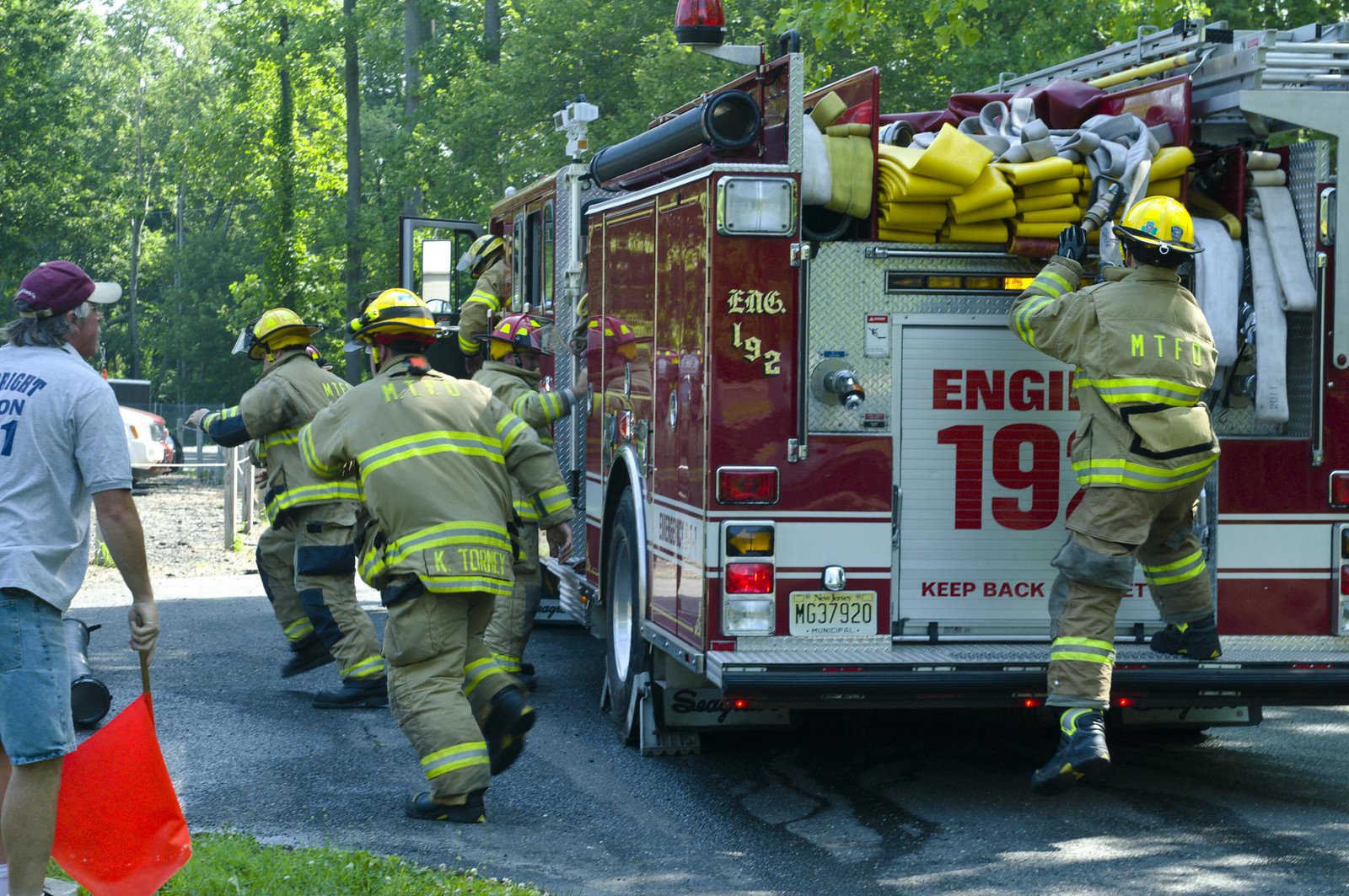The photograph captures a dynamic scene of firefighters swiftly mobilizing from a parked red firetruck on a wet asphalt road in a wooded area. At the back of the firetruck, a fireman with "MTFD" on his uniform is stepping down while pulling a hose. To his left, two firefighters are seen running toward an unseen destination, suggesting a sense of urgency. Beside them, another firefighter is engaged with the side of the truck, possibly retrieving equipment, while further behind, the driver is exiting the cab. In the left corner, a man in a gray shirt and blue shorts, wearing a scarlet baseball cap, holds an orange flag at rest, indicating a training session. The green and yellow-striped uniforms of the firefighters stand out against the forested backdrop, contributing to the overall sense of coordinated action and preparedness.